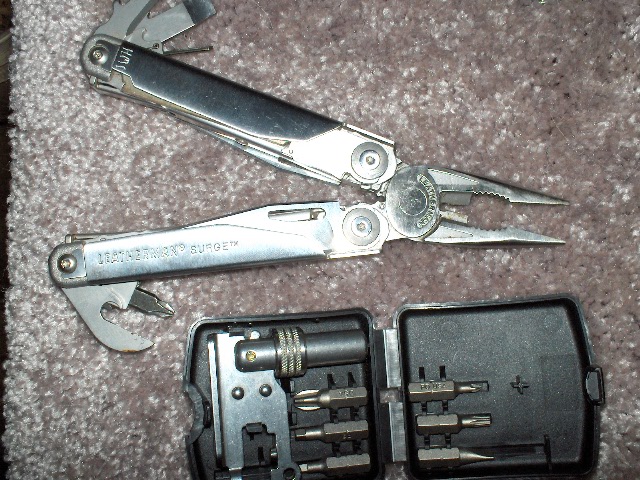The image is an overhead color photograph of a multi-purpose Leatherman style multi-tool, primarily made of stainless steel with some black rubber or plastic grip on one handle. The tool is open, with its plier teeth facing rightward and the handles spread out. Emerging from a rivet at the bottom handle is an array of additional tools such as mini screwdrivers and a bottle opener. Below the multi-tool and partially cut off at the lower right of the image is a black plastic tool case in an open position, revealing various drill and screwdriver bits, including both flathead and crosshead tips. The entire setup rests on a textured surface that varies between descriptions as light brown, dark brown, or grey, featuring a gravelly, stone-like appearance with specks of white throughout.